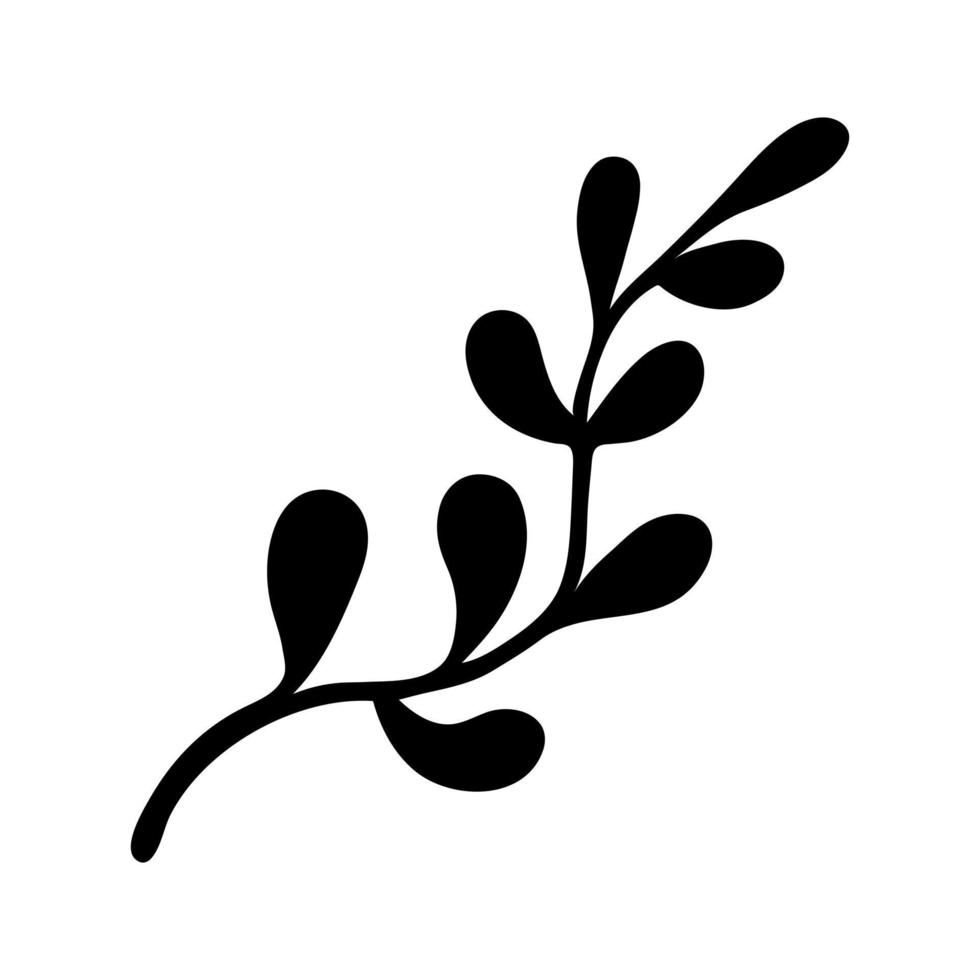The image depicts a minimalist illustration of a plant branch set against a stark white background. The design, rendered in a deep black, features a single, undulating stem that originates in the bottom left corner, curving elegantly upward toward the top right. Along this gently twisting stem, there are teardrop-shaped leaves positioned symmetrically on either side, giving the appearance of an organic vine. The leaves, rounded at their tips, start larger at the base of the stem and progressively decrease in size as they reach upward. The stem similarly tapers, becoming thinner as it ascends. At the very end of the branch, a final, smaller leaf completes the delicate, balanced composition of the artwork.